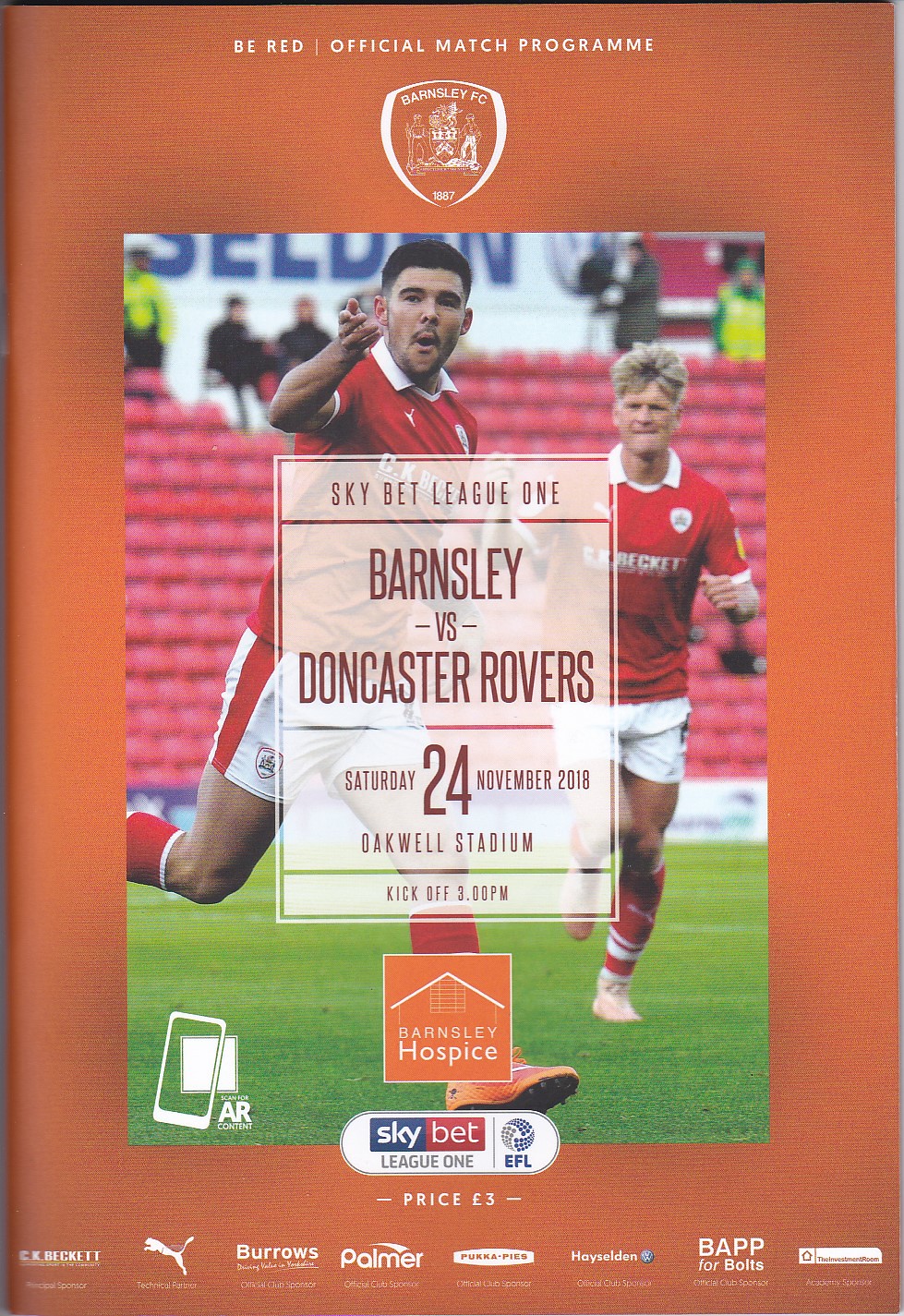The poster features a portrait-oriented layout dominated by a burnt orange background. At the top center, it displays the title "Be Red, Official Match Program" in bold white text. Below this, a white outlined shield contains the emblem for Barnsley FC, established in 1887, featuring two men flanking a central trophy. Central to the design is a large, vivid photograph of two soccer players in motion on a field. Both players don red jerseys with white collars, red knee-high socks, and white shorts with a red stripe. They are set against a backdrop of red spectator seats with several fans visible.

Overlaying the image is a translucent, light tan rectangle with red text announcing "Sky Bet League One: Barnsley vs. Doncaster Rovers, Saturday 24th November 2018, Oakwell Stadium, Kickoff 3:00 PM." Beneath this, an orange square with white text promotes Barnsley Hospice. In the lower left corner, an icon suggests scanning for AR content using a cell phone.

Occupying the bottom center is a pill-shaped oval with the "Sky Bet League One EFL" logo and a note that reads "Price: Three Pounds." A footer along the bottom edge displays multiple sponsor logos, including CK Bennett (technical partner), Puma, Burroughs, Palmer, Pucca Pies, Hayes Seldon, BAPP for Bolts, and The Investment Room.